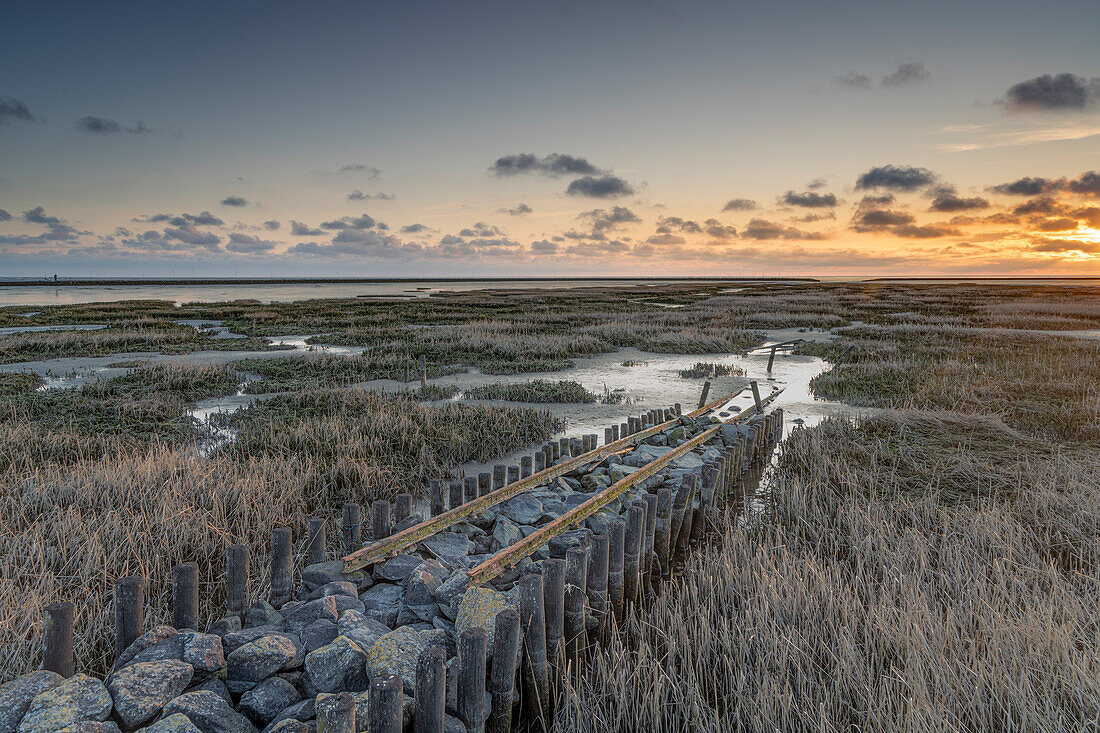A stunning and professionally captured photograph depicts a tranquil coastal marshland at sunrise. The image is bathed in soft, pastel lighting, enhancing its serene and ethereal quality. The foreground features a series of cylindrical wooden posts extending into the shallow water, guiding the viewer's eye towards a central pile of large boulders. Surrounding the posts are patches of dry brush, characteristic of the marshland setting. The sky above is painted in gentle sunrise hues of pink, lavender, and soft blue, blending seamlessly into the overall pastel palette of the scene. The meticulous details and subtle lighting suggest the possibility of digital enhancement, lending an extra layer of beauty to this already captivating landscape.